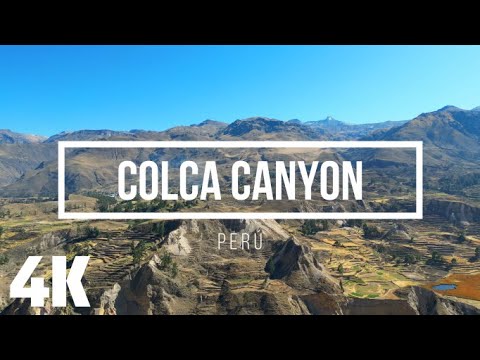This is a high-resolution 4K color photograph of Colca Canyon in Peru, presented within a black rectangular background, emphasizing the image's expansive, wide landscape orientation. The canyon is prominently labeled with "COLCA CANYON" in bold, white capital letters inside a white rectangular box, and beneath it, in smaller text, is the word "PERU." The scene showcases the rugged, brown canyon ridges and arid mountainous terrain, indicative of the dry, high-altitude environment. Green vegetation, including a small pool of water, punctuates the otherwise rocky landscape, while the clear blue sky stretches above. The overall composition hints at possible historical Inca structures within the lower valleys, adding an element of intrigue to the breathtaking natural beauty.